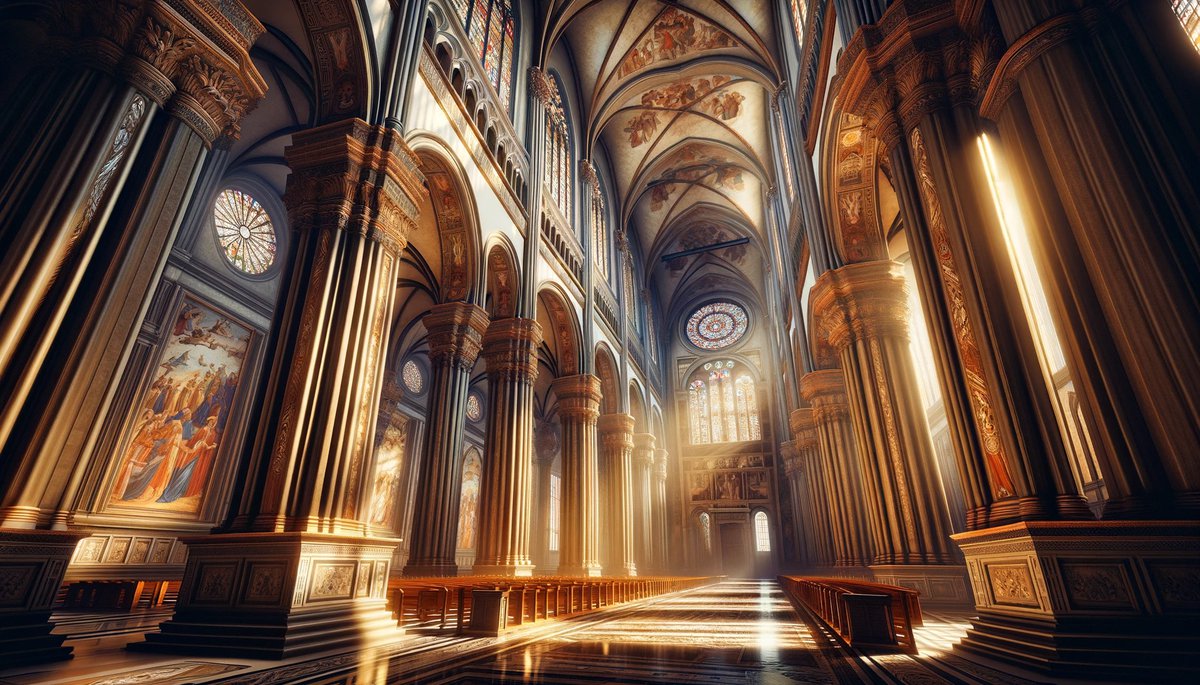The image depicts the interior of a grand, AI-generated cathedral that, while aiming for photorealism, retains a distinct graphical quality. Facing the rear of the church, the viewer is greeted by towering stained glass windows above the entrance, with light streaming through, casting colorful reflections. The walls feature elaborate religious art panels, leading up to an even larger arched window with three main stained glass sections mimicking the window’s shape, and three smaller circular panels at the top. Higher still, an enormous, intricately designed round stained glass window dominates the space. The cathedral features lofty, highly detailed ceilings adorned with murals in shades of beige, brown, and hints of red, evoking a sense of divine grandeur. The floor, likely marble or polished tile, is gleaming and reflects the sunlight filtering through the windows. The church is lined with massive stone columns—seven on the left and five on the right—each embellished with carvings and paintings, showcasing various religious figures. Between the columns on both sides are tall murals and circular stained glass windows. Rows of pews and other seating arrangements are oriented in various directions, some towards the central aisle and others facing the front, further enhancing the sense of intricate design and grand scale that permeates this magnificent virtual cathedral.